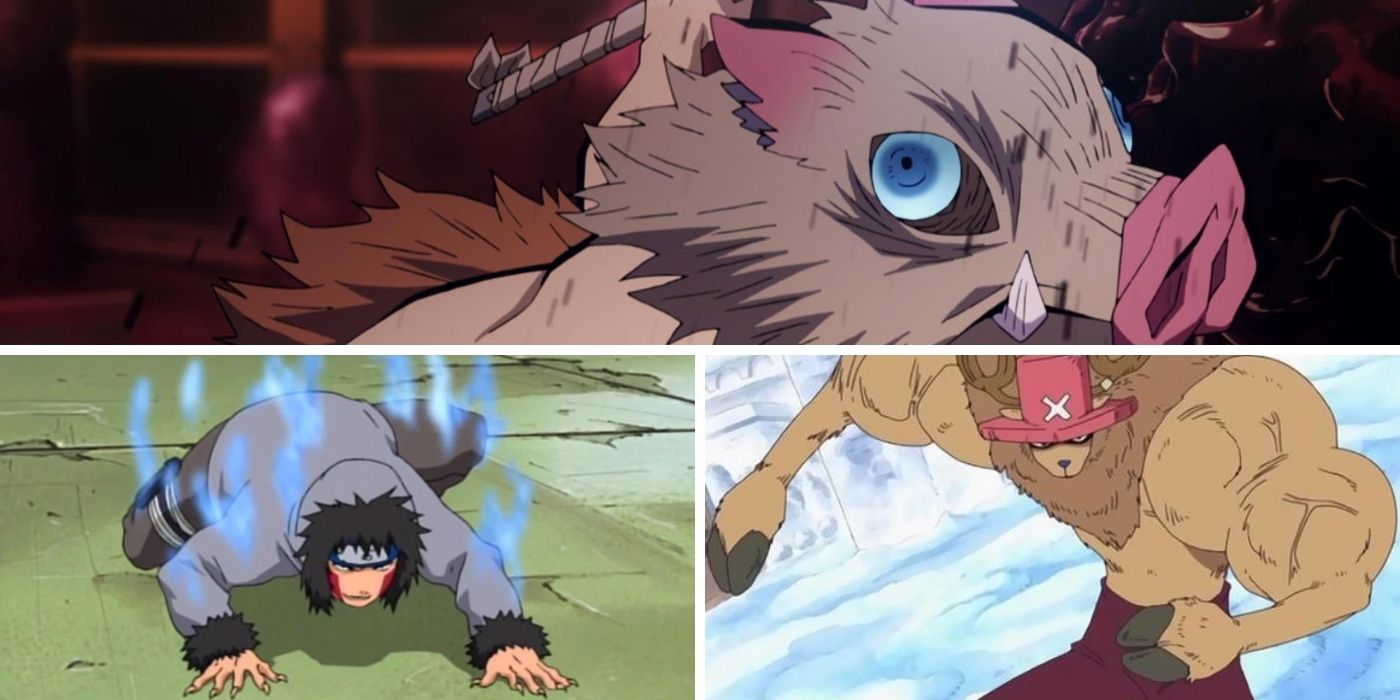The image is a stylized anime collage featuring three distinct characters in separate frames. The largest image at the top is a rectangular depiction of a fearful pig-like creature with a pink snout, pale pink or beige body, pink ears, blue eyes, tusks, and a mane along its back. The bottom left image showcases a man with fur of the same color as the pig, crouching on the ground in a grey hoodie, with a blue light emanating from him. The bottom right image depicts a muscular hybrid creature with a red hat and cloven hooves for hands, standing in an icy setting. This creature has large muscles, a kangaroo-like body, and is wearing maroon-colored pants.